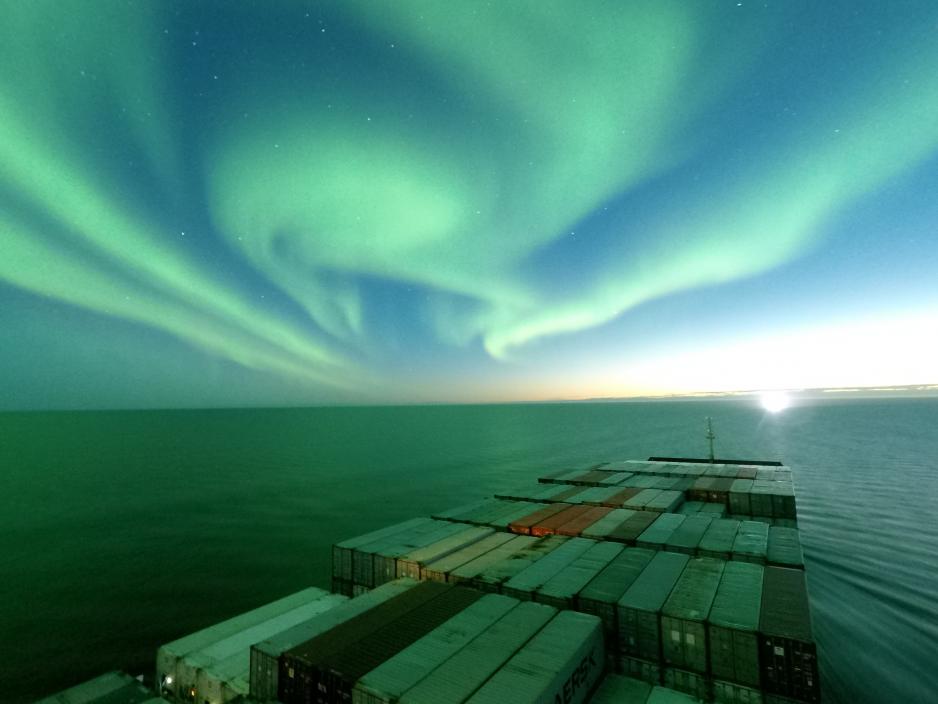The photograph captures an ocean-going cargo ship navigating calm waters under a stunning display of the Aurora Borealis. The color palette is predominantly green and blue, creating a tranquil yet vivid scene. The image is divided into two distinct halves: the bottom third showcases the ship, which appears diagonal in the frame and laden with numerous containers arranged in seven visible rows. The ship is moving towards a bright, white light on the horizon, identified as the setting sun, whose reflection creates a calm, ethereal glow across the water.

Midway through the image, the horizon line is visible, separating the ocean from the sky. Above this line, the sky is a mesmerizing, mint-green canvas adorned with swirling clouds tinged by the Aurora Borealis. Stars dot the sky, enhancing the celestial ambiance. The ship's bow creates gentle waves, adding a sense of movement to the otherwise serene scene. Overall, the photograph beautifully captures the juxtaposition of human industry and the natural wonder of the northern lights.